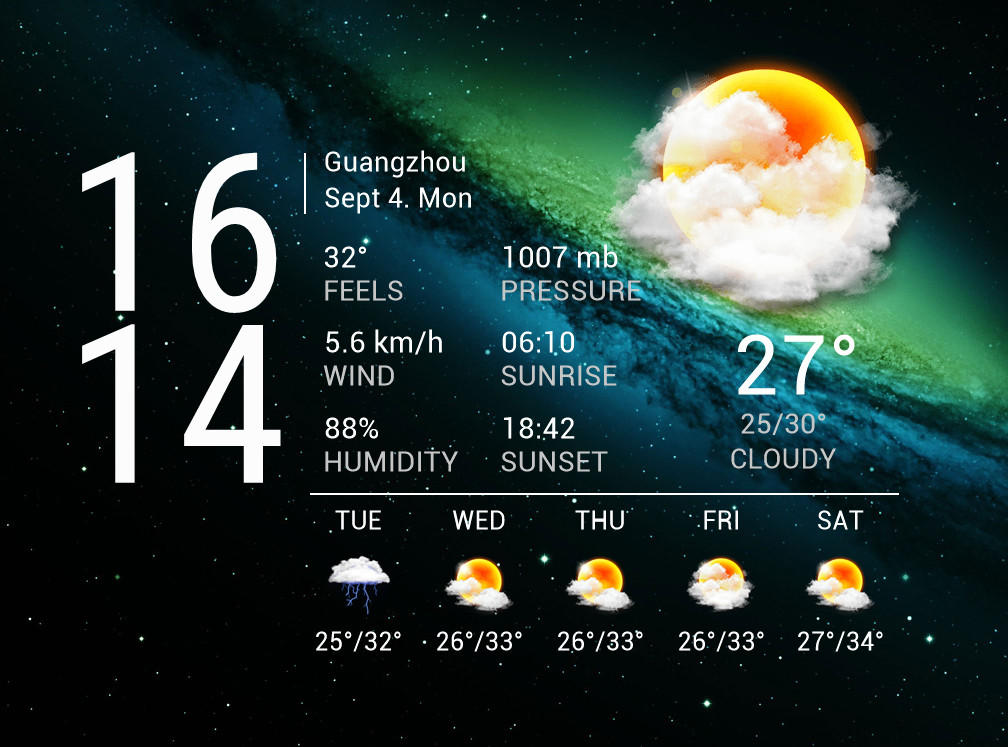In a horizontally rectangular frame, the image appears to be a screenshot from a weather app. The background features a dynamic gradient sky, transitioning from day to night. In the upper right, the sun peeks through clouds against a light blue sky that gradually darkens into an almost black night, dotted with specks representing stars towards the bottom of the frame.

Prominently displayed on the left side are the large white numbers "16" and "14," stacked on top of each other. To the right, it provides detailed weather information for Guangzhou on Monday, September 4th. 

The app's data indicates a 'feels like' temperature of 32 degrees Celsius, atmospheric pressure of 1007 millibars, and a wind speed of 5.6 km/h. The sunrise is recorded at 6:10 AM and the sunset at 6:42 PM. The humidity stands at 88% with the current condition being 27 degrees and cloudy.

Below this, a horizontal bar lists the forecast for the upcoming week – Tuesday, Wednesday, Thursday, Friday, and Saturday – along with the expected high and low temperatures for each day.